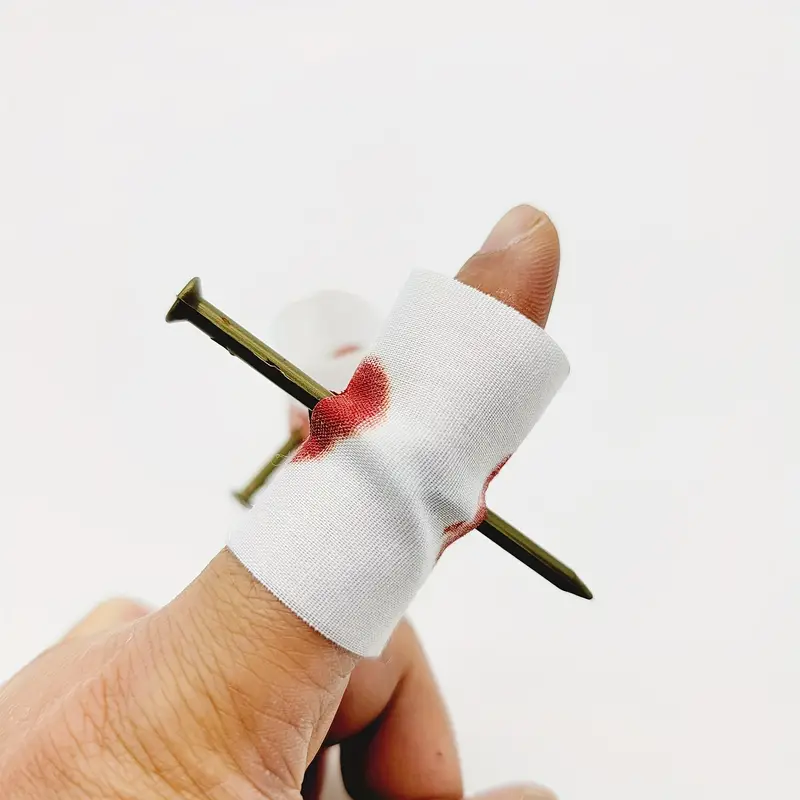The photograph captures a close-up of a person's left index finger, which appears to have sustained a severe and painful injury. The finger, prominently angled from the bottom left to the top right corner of the image, is wrapped in a white gauze bandage. Bloodstains are visible on both the entry and exit points of the wound. A long, grayish-green nail pierces directly through the finger, likely near the knuckle, with one end protruding from the top and the sharpened tip emerging from the bottom. The skin tone of the hand is light, suggesting the person is white, and the fingernail is neatly trimmed. The background of the image is a solid, very light gray, almost white, which enhances the stark details of the injury. Wrinkles are visible on the finger's skin, adding to the realism and intensity of the scene.